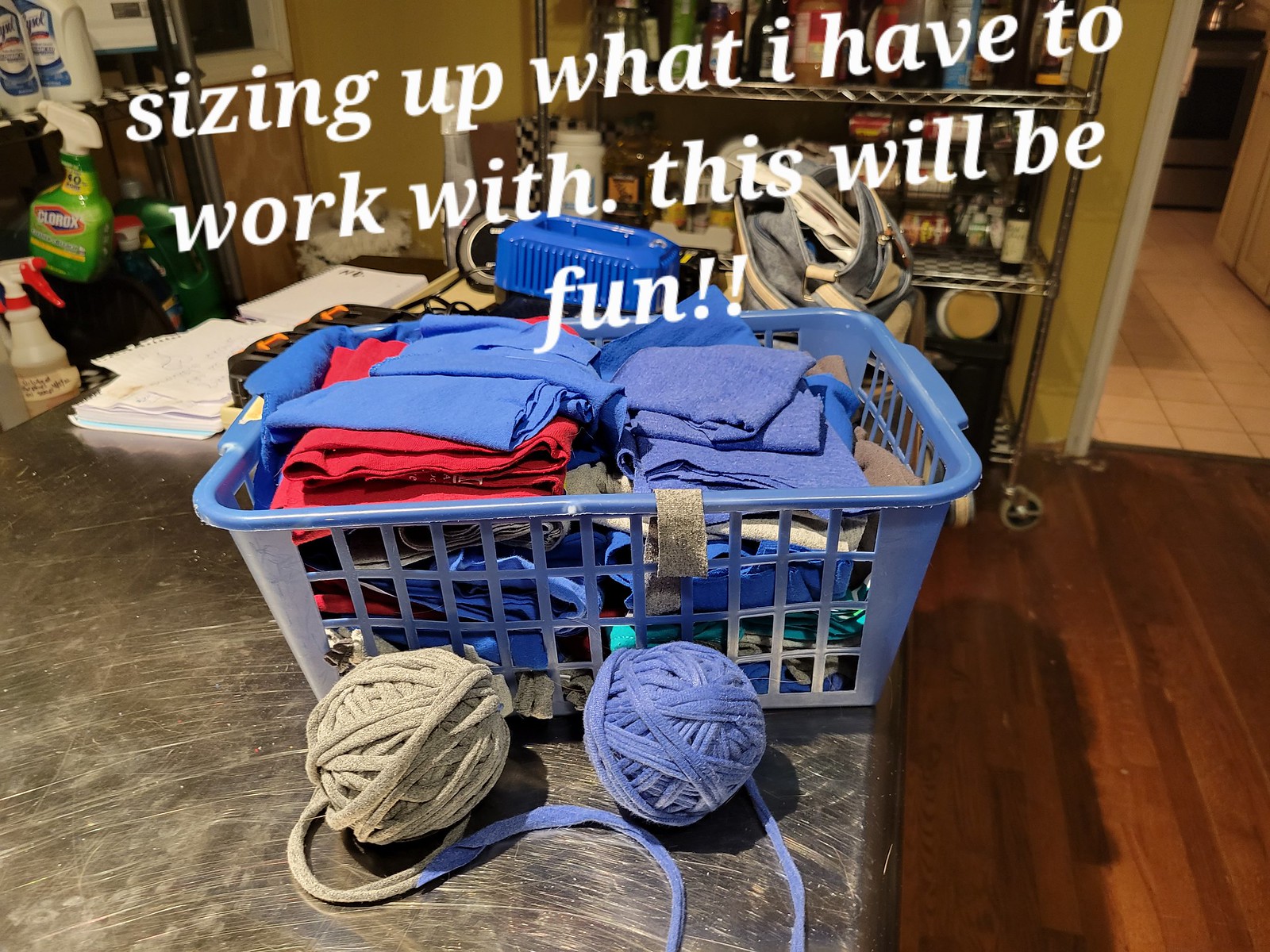In this photograph, the focal point is a light powder blue plastic laundry basket filled with neatly folded clothes, primarily in shades of navy or powder blue and red. The basket is placed on a black table or shelf. In front of it, there are two balls of yarn, one in a matching powder blue and the other in a brownish-gray color. The tabletop also holds various other items including stacks of paper and additional clothing. In the background, the room features brown wooden flooring and metal shelves against the back and left walls. The left shelf holds cleaning supplies, notably bottles of Clorox and Lysol, while the back shelf hosts a variety of items including more bottles. Text at the top of the photo, written in white, reads, "Sizing up what I have to work with. This will be fun."